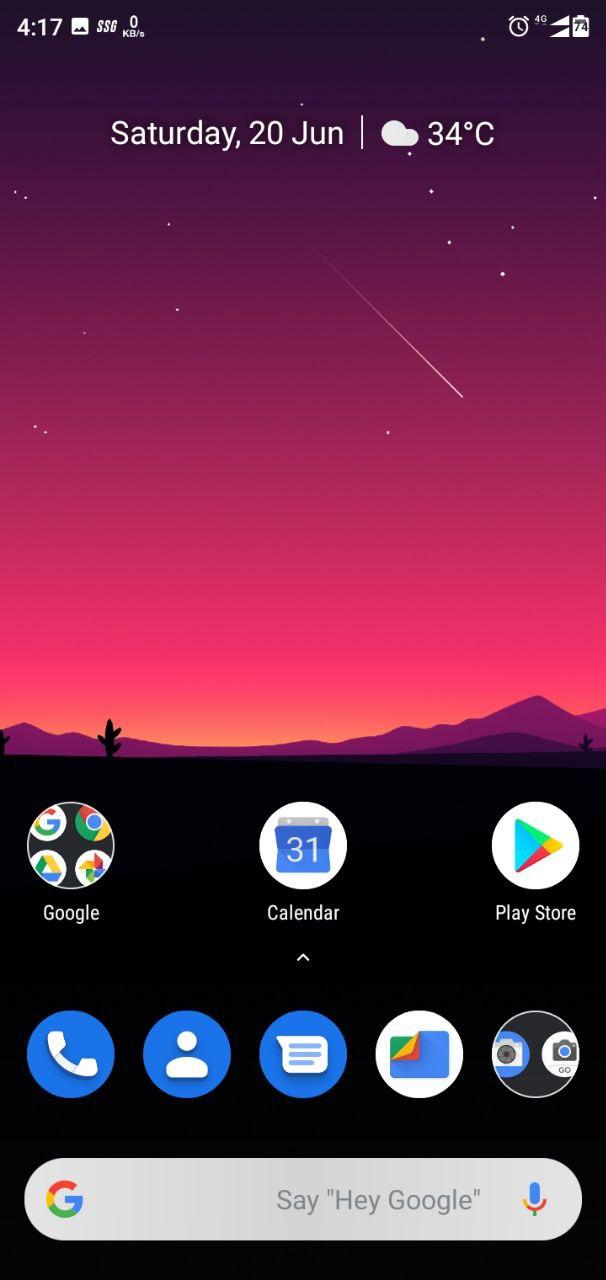This captivating image, likely a screenshot from an Android phone, features a beautifully painted background showcasing a stunning sunrise or sunset. The sky is awash with hues of pink, red, and vibrant yellow-orange, fading into a calming blue, setting the scene behind a silhouette of mountains and black cacti. A scattering of stars and a prominent shooting star streaking from left to right add a touch of celestial magic.

At the top of the screen in white text, the time is displayed as 4:16, with the Instagram app open in the background. Symbols including dollar signs and a bitrate indicator (unfortunately showing zero) are visible. On the right side, notification icons display an alarm clock, 4G connectivity, two different cell service signals, and a battery indicator at 74%. The date is marked as Saturday, June 20th, with the weather noted as cloudy and a sweltering 34°C.

The bottom part of the screen is populated with various app icons. Three black circular icons represent Google, Calendar, and the Play Store. Further down, there are icons for the phone, contacts, text messages, documents, and two different camera functions. Additionally, a gray search bar at the bottom invites users to "Say 'Hey Google'."

Overall, this detailed and intricately depicted screenshot highlights the artistic background and the functional interface of an Android device.